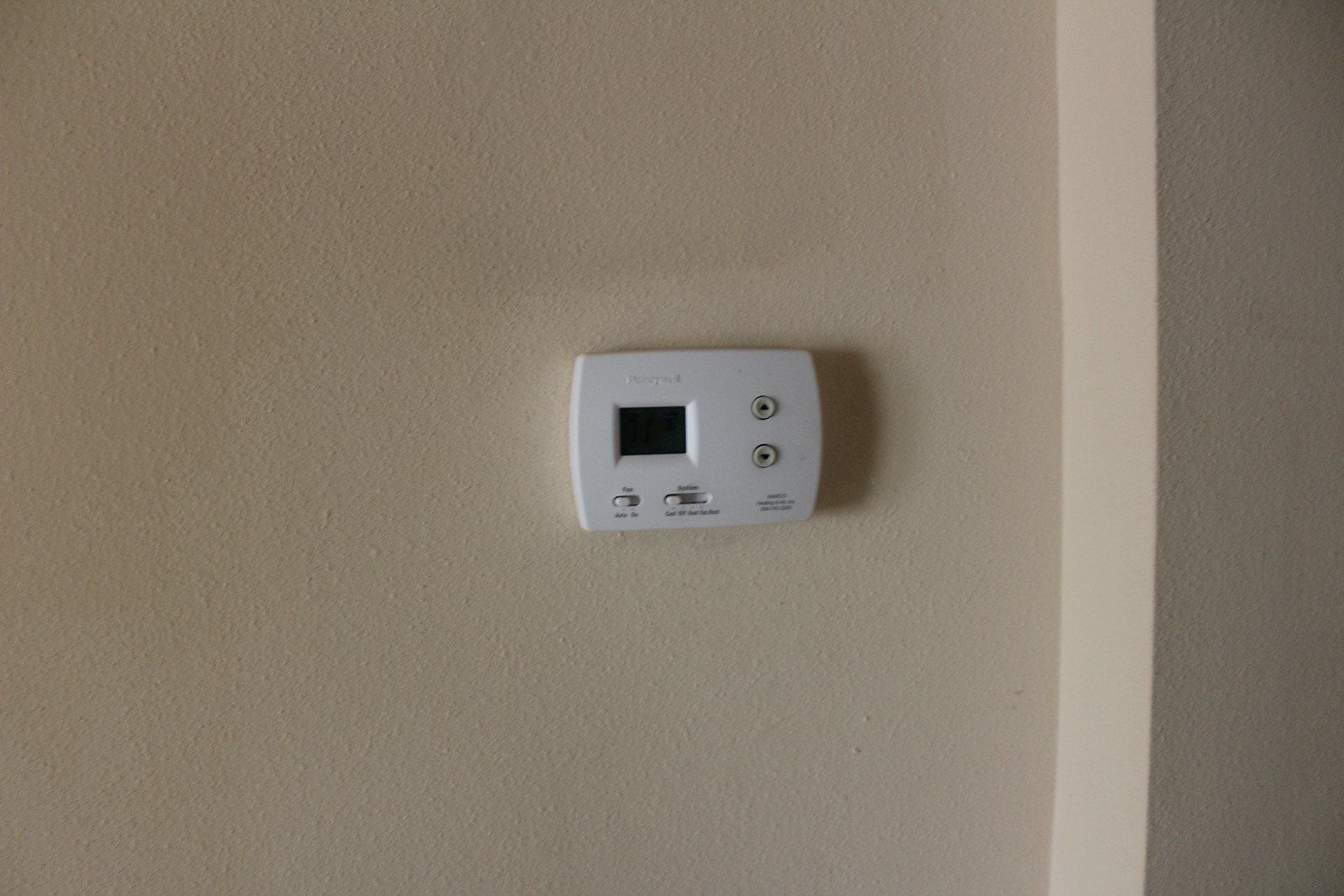The image features a white Honeywell thermostat that seems to date back to the 2000s. The device has a compact, rectangular shape with a simple design. It is mounted on a peach-colored wall, which has a slight indentation behind the thermostat, possibly indicating a storage space for wiring.

The thermostat includes a small screen located centrally on the left side, which is an older type that only lights up when a button is pressed. The screen remains a dark gray-green color until activated. Above the screen, "Honeywell" is printed in small white letters.

On the right side of the thermostat, there are two small white buttons with black text, marked with up and down arrows for adjusting the temperature. In the bottom right corner of the device, there is some text that is not legible.

The thermostat is equipped with two knobs at the bottom. The left knob allows users to toggle between 'Auto' and 'On' settings, offering the choice of automatic regulation or manual control. The right knob provides options for 'Off', 'Heat', and 'Cool', enabling users to set the thermostat to heat, cool, or turn off the system entirely. This configuration allows for flexible management of heating and cooling based on different needs and conditions.